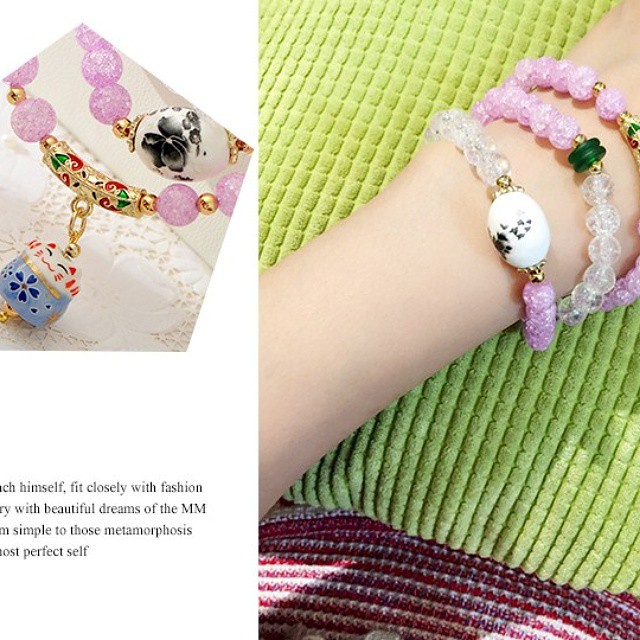The image shows a detailed composition featuring a person's lap, which serves as the backdrop for a series of intricate objects. The bottom part of the image reveals a portion of their shirt and potentially a pillow resting on their lap. Extending across the image from the right side is an arm adorned with multiple bracelets. These bracelets are predominantly beaded, featuring pink and transparent crystal-like beads, interspersed with pendant-like elements that may include gold pieces or unique shaped beads such as a large white one and a small green one.

On the left side of the image, near the top, there is a close-up of one of these bracelets, possibly highlighting its detailed artisanry. This depiction includes miniature pink bubbles and a blue cat figurine, suggesting a handmade and intricate jewelry design. 

Additionally, there is partially obscured text in the bottom left corner that reads, "Ick himself fit closely with fashion, with beautiful dreams of the M.M., simple to see those metamorphose, most perfect self." The setting or style of the image indicates a showcase for these pieces of jewelry, capturing their craftsmanship and the harmonious blend of colors including white, black, light blue, dark blue, tan, green, red, gold, pink, gray, light green, and maroon.